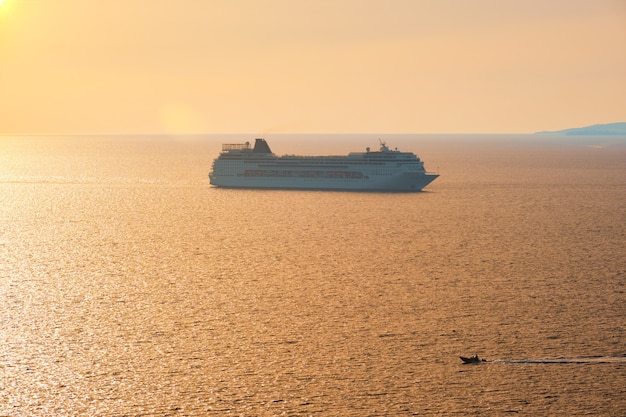In this detailed and vivid image, a large cruise ship dominates the upper half of the scene as it sails through the open ocean at sunset. The ship, casting a bluish shadow in the soft day-end light, faces toward the right side of the frame. The overall palette of the photograph is bathed in a warm gradient of peach, orange, and golden hues, which lends a hazy, almost ethereal quality to the image. 

The sky, transitioning from yellow to pink to purple and finally bluish near the horizon, reflects these colors back onto the calm water. To the right, a distant mountain or hill offers a serene backdrop to the tranquil scene.

In striking contrast to the imposing cruise ship, a tiny speedboat, almost silhouetted and appearing nearly black, cuts through the water in the foreground, leaving a visible trail of ripples behind it as it heads towards the left. The sun, although not fully visible, peeks slightly from the top left corner, illuminating this picturesque maritime landscape.